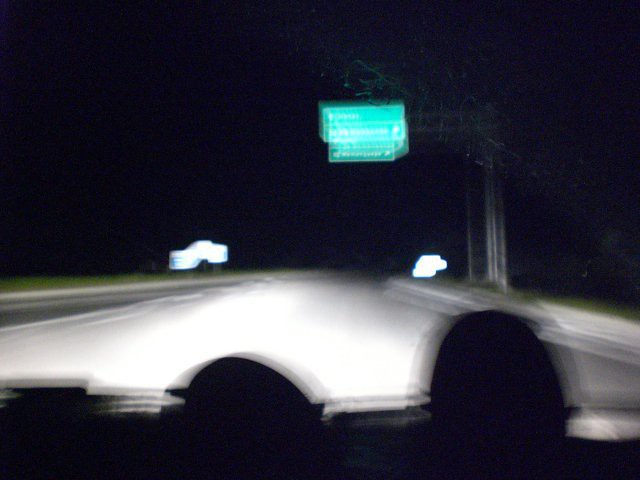This is a blurry nighttime photograph taken from inside a moving vehicle, looking through the windshield as the car drives down a highway. In the foreground, the black outline of the dashboard is visible, including the faint outlines of windshield wipers, a half-circle with a ring around it, and a dark black oval to the right. The road, which appears white, reflects the car's headlights and fades into the distance. On the right side of the road, a blurry silver guardrail can be seen. On either side of the image, green grass is faintly illuminated by the car's headlights. To the left of the road, there is a light-colored curb accompanied by patches of grass. Mounted on metal poles ahead, green highway exit signs with white writing are visible, with one sign reflecting light faintly in the distance. The photograph captures the indistinct shapes and reflective surfaces typical of a night drive, with the overall scene shrouded in darkness.